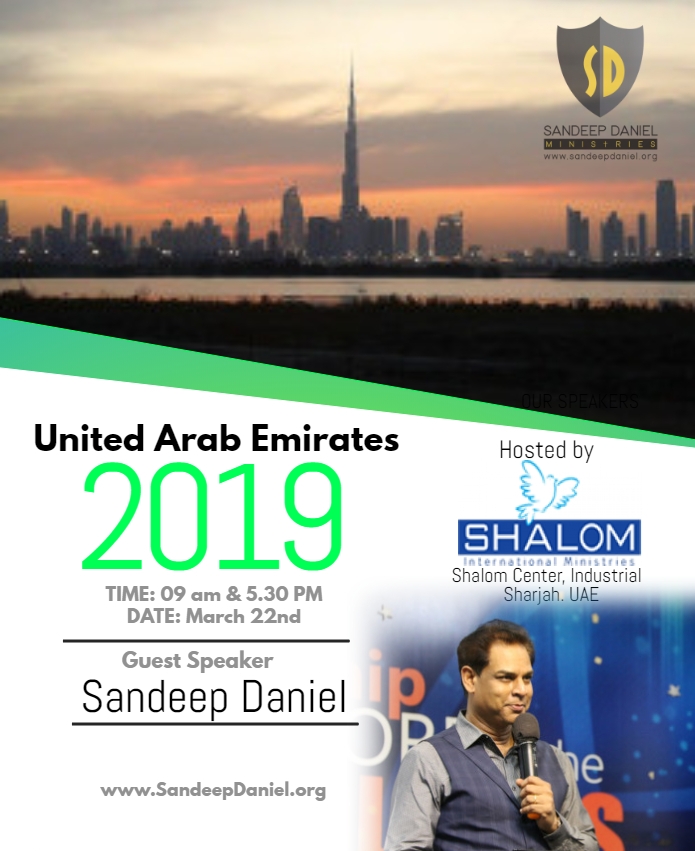The promotional image is for an event in the United Arab Emirates taking place in 2019. The top half of the image showcases a picturesque cityscape, viewed from across a large body of water. Dominating the skyline is an exceptionally tall tower, much taller than the other buildings, which resembles a spike piercing the sky. The scene captures a dramatic sunset, with streaks of red and orange intermingled with white and gray clouds against the darkening sky. The foreground features dark, bushy areas suggesting some foliage. In the top right corner, there's a gray SHIELD logo with the letters "SD" and the text "Sandeep Daniel miniseries www.sandeepdaniel.org."

The bottom half of the image contains multiple lines of text on a white background. Boldly stated in bright green are the words "United Arab Emirates 2019." Below that, in black text, it reads "time 09:00 a.m. and 5:30 p.m., date March 22nd." Further down, it announces "Guest speaker Sandeep Daniel www.sandeepdaniel.org," followed by "hosted by Shalom International Ministries Shalom Center, Industrial Sarja, UAE." On the bottom right, there's a photograph of Sandeep Daniel. He is depicted speaking into a microphone, wearing a gray vest over a shirt, and set against a blue background.